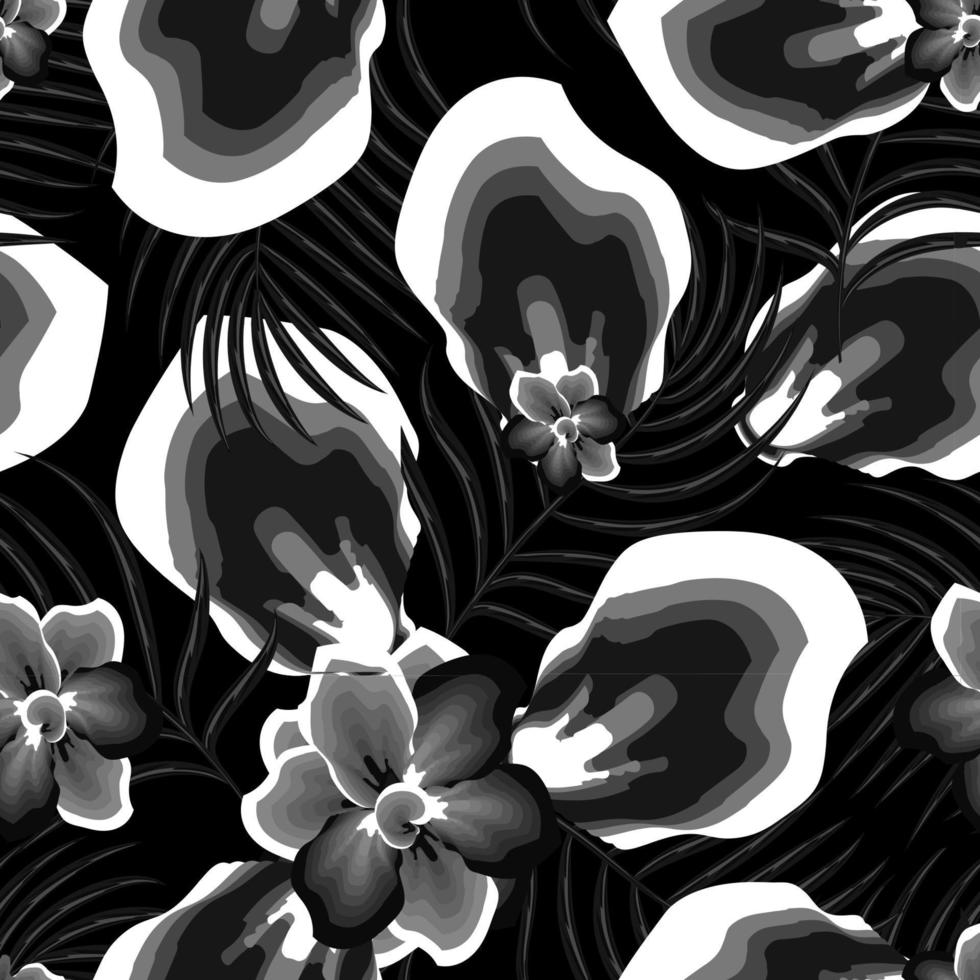This black and white graphic design features a repeating pattern of Hawaiian-inspired flowers and leaves. The monochromatic artwork employs shades of white, light gray, dark gray, and black to create depth and contrast. The floral elements are positioned in various orientations, with some flowers and leaves pointing left, right, or situated upside down, adding a dynamic feel to the design. The palm fronds and leafy shapes in the pattern show subtle hints of gray on the otherwise black surfaces. This illustration has a distinctive, repetitive layout, making it suitable for tiling as a seamless background. The composition is devoid of any text, people, or animals, emphasizing its purely ornamental and decorative nature.